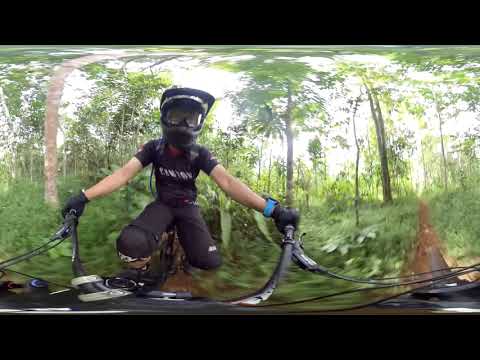In a vivid 360-degree panoramic image, the close-up shows a person of indeterminate gender, clad entirely in black gear, riding what appears to be a bicycle or dirt bike through a dense, green forest. The individual is equipped with a black helmet and goggles, obscuring their face, and black gloves. They wear a shirt with white writing and a blue watch or wristband on their arm. Their legs are bent, indicating their feet are on the pedals, and they grip the black handlebars firmly. The surrounding environment is rich with trees, bushes, and shrubbery, creating a lush, wooded setting. There are visible paths on both sides: one directly behind them and another, well-worn dirt path with no grass, to the right. The sky peeks through the treetops, appearing bright and almost glaring white. The scene is bordered by a thick black stripe at the top and bottom of the image.